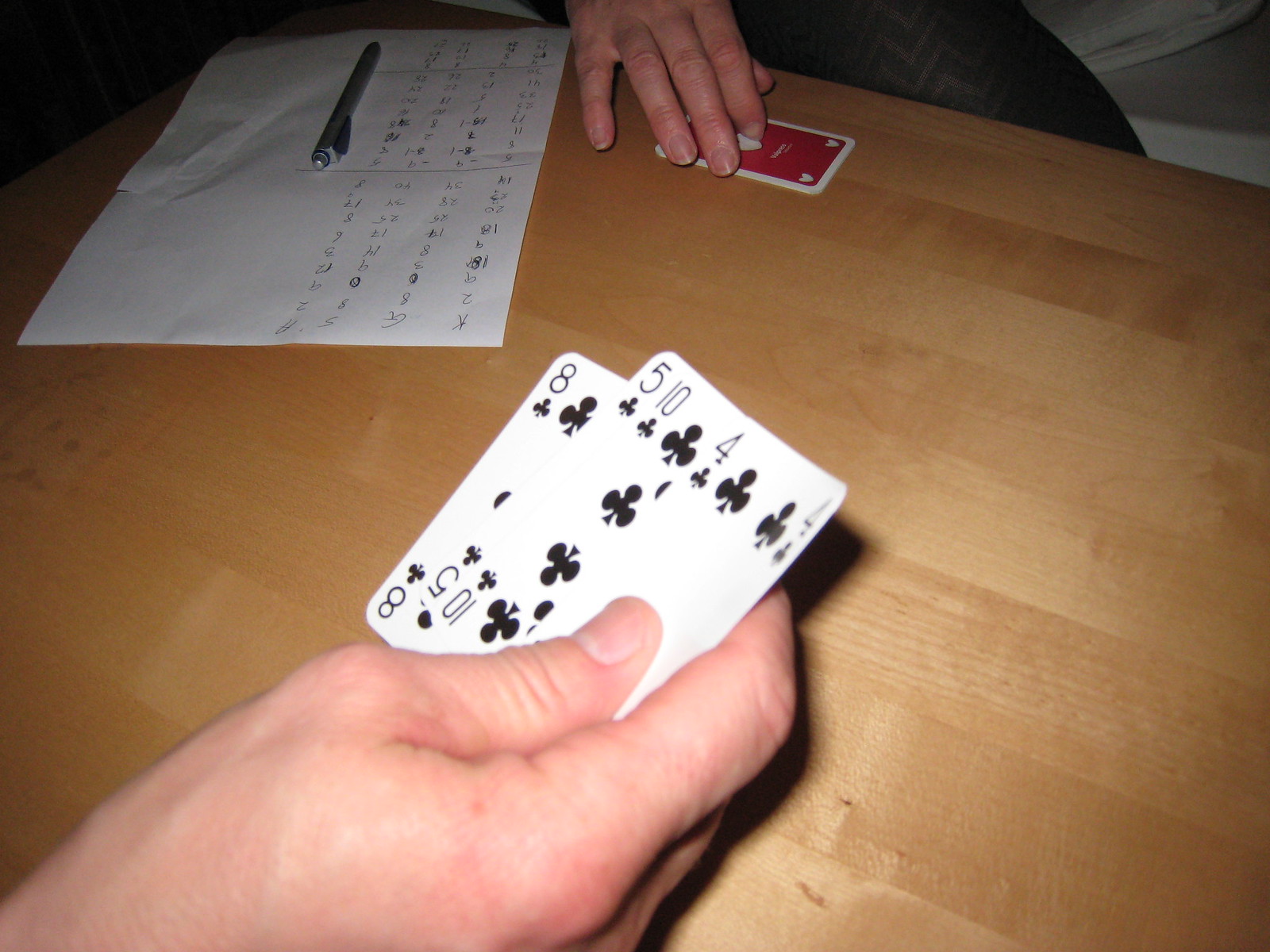In the image, two individuals are engaged in a card game at a wooden table. The table, which is square and slightly oriented towards the top left corner of the image, exhibits a surface that is mostly smooth but shows some signs of wear. A piece of white paper lies on the table, with a gray pen resting atop it. The paper appears to be a score sheet, featuring four vertical columns filled with numbers, indicating ongoing scorekeeping.

One player's hand, positioned near the top of the image, is partially visible. This player is seated on a gray couch and is clad in gray pants, a portion of which is observable. Their hand covers some red playing cards adorned with white hearts on the back. Another hand, belonging to the second player, emerges from the bottom left corner of the image, holding four cards. From top to bottom (right to left), these cards are the four of clubs, ten of clubs, five of clubs, and eight of clubs. The overall setting conveys a cozy and engaged atmosphere focused on the card game.